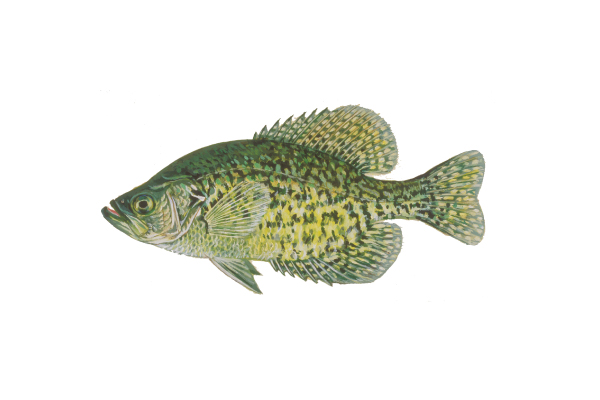This is an illustration of a fish on a white background, likely intended to depict a fish for a book or educational purposes. The fish's body is predominantly green, transitioning from a darker green near the head to a lighter, yellowish-cream color under its chin and speckled with black, yellow, and gold spots. The side profile highlights the fish's pointed face and slightly open mouth, with a texture that adds depth to its appearance. Its spade-shaped body features prominent dorsal and ventral fins that mirror each other in color, with partially serrated edges that round off smoothly. The rounded, arrowhead-like tail fin complements the body’s coloration, which is consistent throughout. The fish’s eye is detailed with shades of yellow and green, adding to its realistic depiction. The overall shape is reminiscent of a guppy or a young grouper, making it a stereotypical fish image distinguished by its distinctive, detailed presentation.